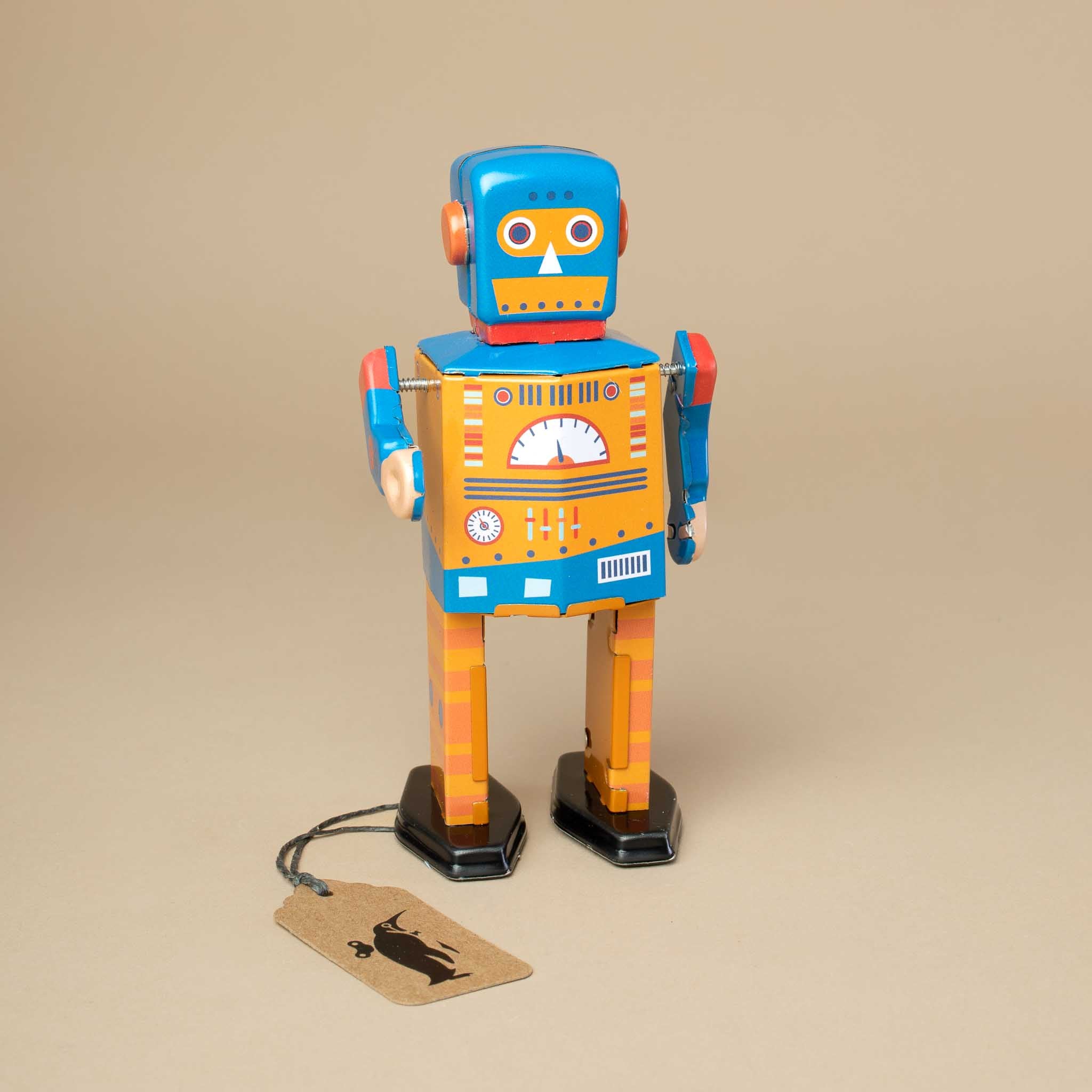This image portrays a vintage-style toy robot, possibly a handcrafted item or one put up for sale, positioned against a beige backdrop. The robot, primarily in shades of light and dark orange with blue accents, stands upright on a desk or platform. Its head, square and blue, features a white nose, while its square-shaped body is adorned with various drawn-on controls, dials, and buttons. The blue arms are attached with screws, and its small metal legs culminate in black base plates for stability. Notably, a brown tag affixed with gray rope dangles from the robot's left leg, showcasing an illustration of a penguin with a wind-up mechanism on its back. The entire scene is set within a light brown background.